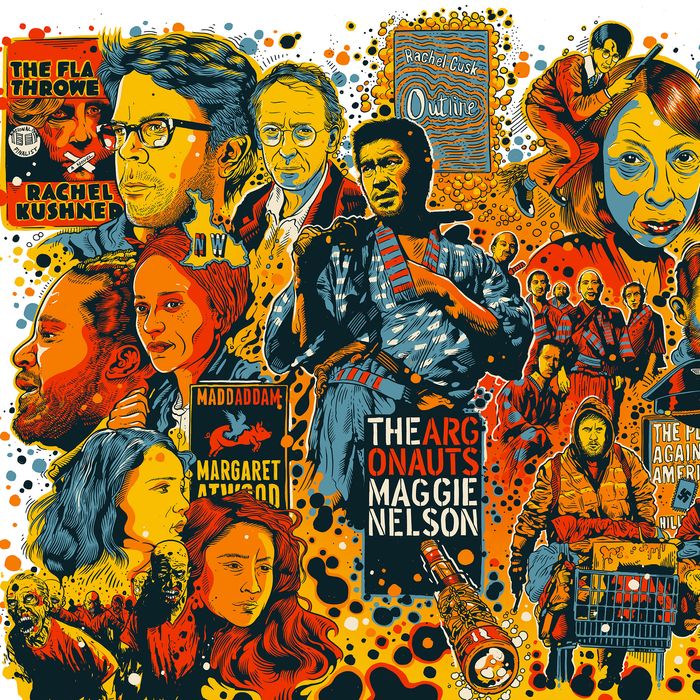The image is an intricate, colorful collage featuring an assortment of figures, predominantly rendered in orange-yellow hues with touches of blue shading. Prominently, a group of Chinese men are depicted in traditional robes, their heads appearing to overshadow one another. Interspersed among them are close-up portraits of women’s faces, and various other characters, some resembling comic book figures. Lower in the composition, a horde of zombie-like figures in t-shirts adds a surreal touch. The central text reads "The Argonauts, Maggie Nelson," while other textual elements include signs for "Madame Margaret" and "Throw Rachel Kuscht." The collage is dotted with round, bubble-like circles, and movie posters with minimalist design occupy parts of the image. One notable figure, dressed in red, white, and blue robes, appears ready for combat, and another in the bottom right is pushing a shopping cart, suggesting homelessness. The overall effect of the collage, filled with overlapping, stylized faces, evokes a sense of chaos and melancholy.